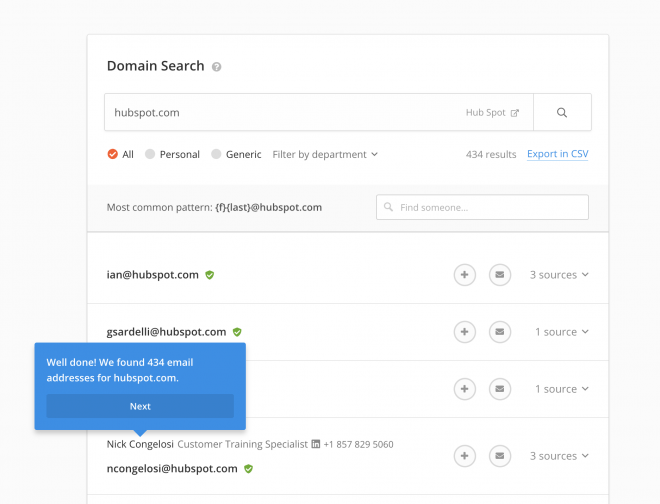On the website designed for domain searches, the interface features a light gray background. Dominating the page is a large white box divided into several components. 

In the top left corner of this white box, the bold text "Domain Search" is displayed with a question mark icon to its right. Below this title, there is a search bar where "HubSpot.com" has been typed. To the right, a faded icon with the label "HubSpot" is noticeable. Adjacent to the search bar is a search button featuring a magnifying glass icon.

Below this section, are several radio buttons, each with different options. From left to right, the options are "All" (selected, indicating an orange checkmark), "Personal," and "Generic." Further right, there's a "Filter by Department" drop-down menu, next to a section that displays "433 results" and offers a link to export these results in CSV format.

Directly beneath there is a gray banner that reads "Most Common Pattern" with an example email format "last@HubSpot.com." To the right of this banner is a white search bar containing a magnifying glass icon and the text "Find someone..."

Below the banner are four rows of results. The first two rows display "IAN@HubSpot.com" and "GSRValley@HubSpot.com," each with a green verification check mark. To the right, there are icons for adding as a contact and sending an email, along with a drop-down menu showing the number of sources.

The third row is partly obscured by a blue pop-up box that says, "Well done, we found 434 email addresses for HubSpot.com," with a darker blue button labeled "Next" at the bottom. This pop-up points towards the last row.

In the fourth row, the name "Nick Congonacci" is displayed with the title "Customer Training Specialist." Next to an Indeed icon and a phone number, Nick's HubSpot email address is also listed.